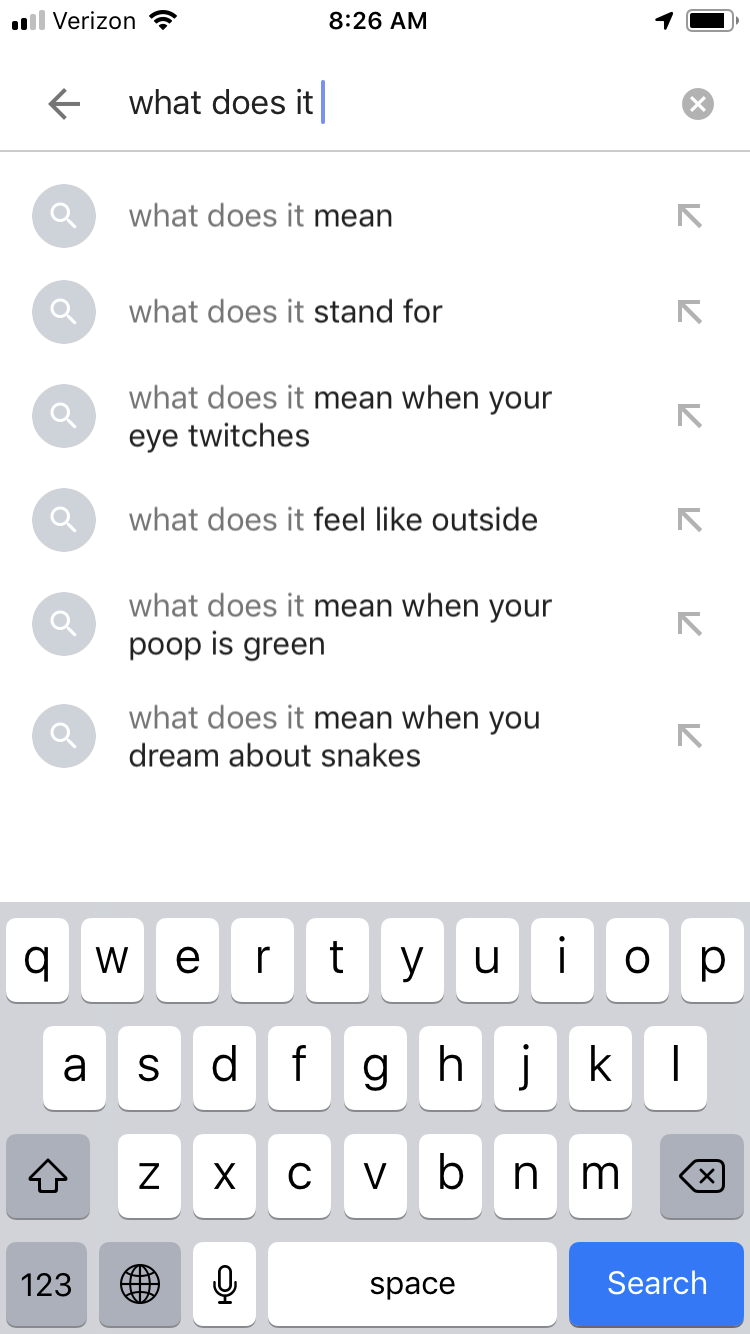A detailed screenshot from a smartphone displays various elements on a white background. In the upper left-hand corner, black text indicates the cell phone service strength, accompanied by the word "Verizon" and the Wi-Fi signal strength icon. Centered at the top is the time, which reads 8:26 AM. In the upper right-hand corner, the battery percentage is shown alongside a location icon, suggesting location services are active.

Beneath the timestamp, there appears to be a search interface that closely resembles a Google search bar but seems to be an internal phone search function instead. On the left-hand side, an arrow points left, implying a back navigation option. The typed query reads, "what does it?" and immediately below, six auto-complete search suggestions are listed:

1. "What does it mean?"
2. "What does it stand for?"
3. "What does it mean when your eye twitches?"
4. "What does it feel like outside?"
5. "What does it mean when your poop is green?"
6. "What does it mean when you dream about snakes?"

At the bottom of the screen, a keyboard is displayed, indicating that the user can continue typing their search query. The overall image captures a moment of curiosity and the subsequent suggestions provided by the phone's search function.